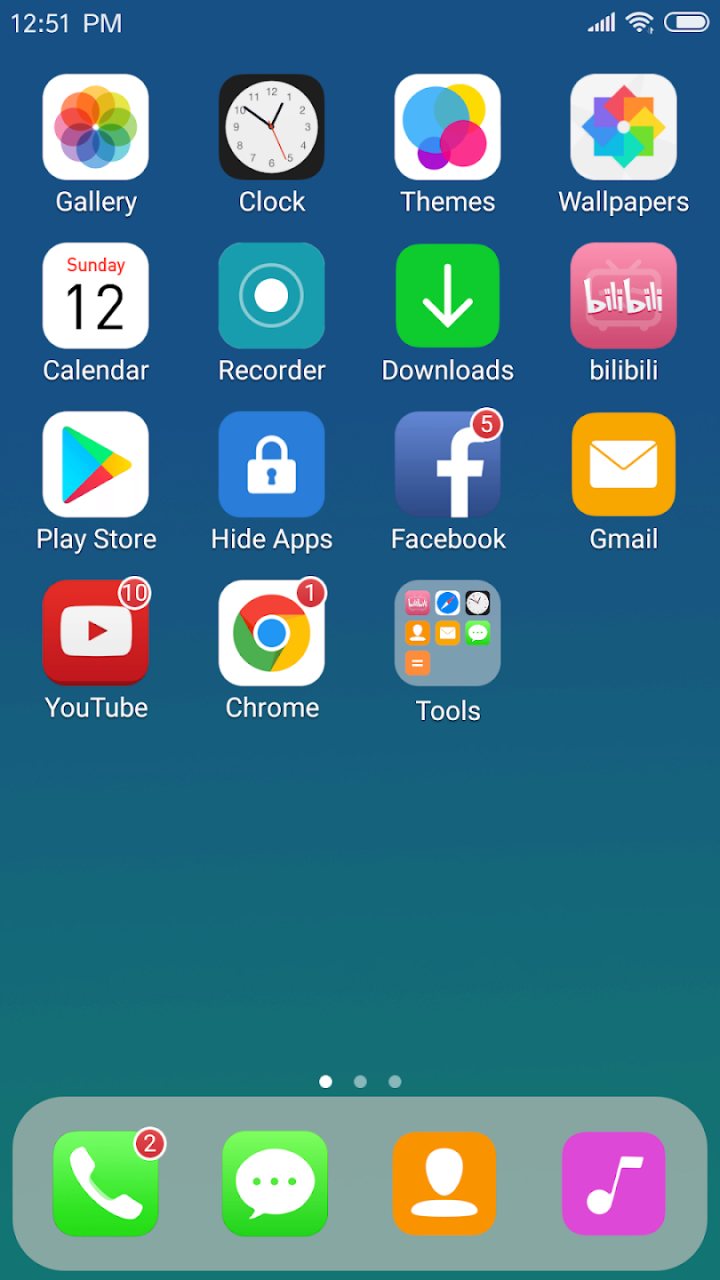The screenshot displays the home screen of an iPhone at 12:51 PM, showcasing a neatly organized grid of app icons. The top section features 19 icons arranged in four rows.

In the first row, from left to right, the icons are:
1. Google Photos (Gallery)
2. Clock
3. Themes
4. Wallpapers

The second row includes:
1. Calendar
2. Recorder
3. Downloads
4. Bilibili

The third row features:
1. Play Store
2. Hot Apps
3. Facebook
4. Gmail

In the fourth row, there are:
1. YouTube
2. Chrome
3. Tools

Note that the fourth row has only three icons, leaving the last spot empty. 

At the bottom of the screen, the dock holds four frequently used apps:
1. Phone (indicating two missed calls or notifications)
2. Messages (indicating new messages)
3. Contacts (represented by an orange icon with a silhouette)
4. Music (indicated by a purple icon with a white musical note)

This detailed layout provides a glimpse into the user's app preferences and current notifications.